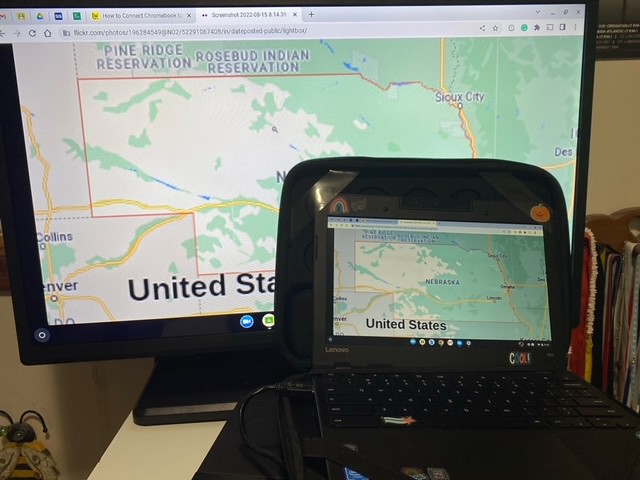In this image, a black laptop is positioned in the bottom right-hand quadrant, open inside a laptop bag of the same color. The laptop is plugged in, indicated by the visible charging cable. Both the laptop screen and a larger external monitor behind it display the same image of the state of Nebraska, taken from a Google Maps-like application. The map highlights the Pine Ridge Reservation and Rosebud Indian Reservation, with the words “United States” appearing prominently in large black letters. The map features green and beige hues with yellow lines signifying major U.S. highways. In the background, a grayish wall is visible, accompanied by a neatly arranged row of books in the bottom right corner and a yellow, bee-like object in the bottom left corner.